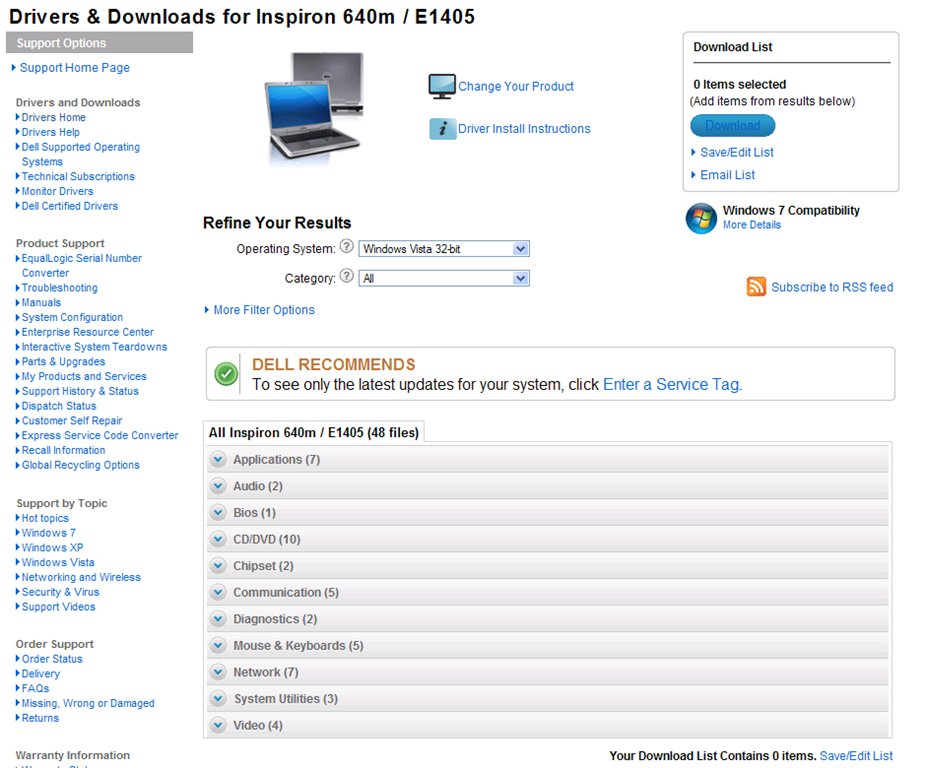The top section of the image contains the heading "Drivers and Downloads for Enspiron 640M-E1405" in black text on the left side. Beneath this is a grey rectangle with illegible text. Below the grey rectangle, there's a sequence of right-pointing arrows interspersed with blue and black text, continuing downwards in a consistent pattern: arrow, blue text, black text, and so forth.

On the right side, towards the top, is an image depicting two laptops, one facing forward and the other backward. Adjacent to this image is a small computer screen icon with the text "Change your product" beside it. Below this, there is a blue rectangle containing a cursive 'i', labeled "Driver Install Instructions." Following this is a grey-outlined rectangle titled "Download List," indicating zero items selected with a note in parentheses reading "Add items from results below." A blue button nearby has some text in darker blue that is not legible, accompanied by right-pointing arrows labeled "Save/Edit List" and "Email List."

Underneath the laptop images is a section titled "Refine your results," which includes options for "Operating System" with a question mark icon inside a circle and an unreadable white rectangle, followed by a light blue square with a downward arrow. The next category is "Category," also marked with a question mark inside a circle, an unreadable white rectangle, and another blue square with a downward arrow.

Further down, there is another grey-outlined rectangle containing a green circle with a checkmark and a statement next to it: "Dell recommends that to see only the latest updates for your system click enter a service tag." Below this is a white rectangle with some obscured writing.

On the left-hand side of the image, aligned vertically, is a series of grey rectangles with downward-pointing arrows on circles to their left and text on their right.

Returning to the top, under the download list section, there's a Windows logo beside text indicating "Windows 7 compatibility more details," followed by an orange WiFi symbol and some unreadable text. At the very bottom, there are black text and blue text, which are also unreadable.